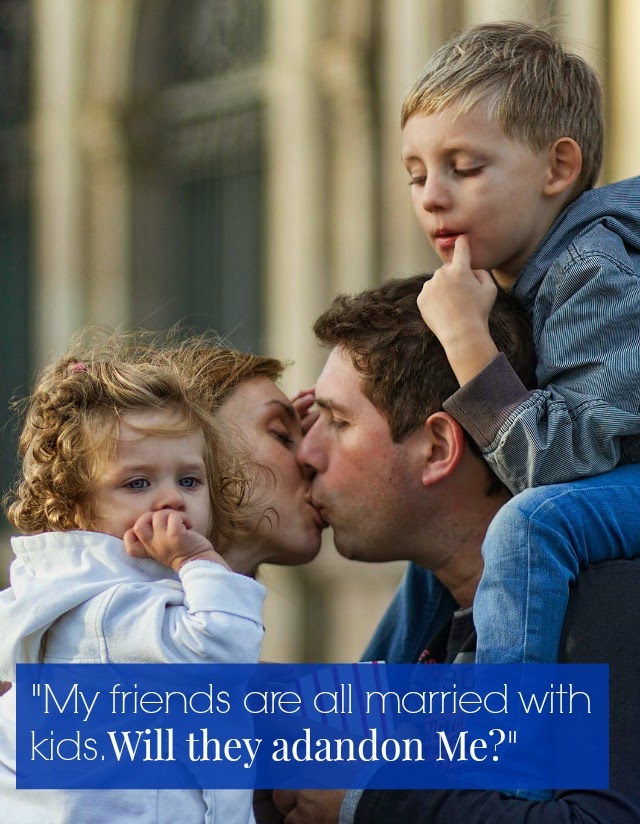In the image, a Caucasian family is captured in a candid moment. On the left, a mother with blonde hair is kissing a man with medium-length brown hair, presumably her husband. The woman is holding a little girl with blonde, curly hair who is sucking her thumb. The girl is wearing a white hooded jacket. On the right, the man, dressed in a gray jacket, has a little boy on his shoulders. The boy, with short blonde hair, is looking down with his left forefinger at the corner of his mouth. He is dressed in a grayish-green hoodie and blue jeans. The background reveals a tan, columned building with an arched entryway and blurry, smoky-colored windows, suggesting an urban setting. Overlaying the bottom of the image is a blue rectangle with the white text: "My friends are all married with kids. Will they abandon me?"